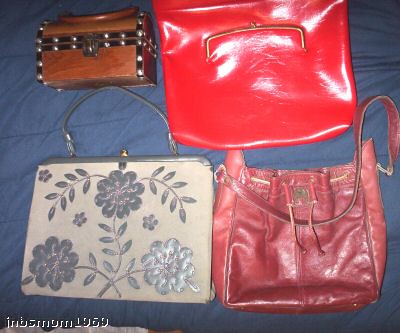The image showcases four distinct purses arrayed on a dark blue bedspread, illuminated by a camera flash. A watermark at the lower left reads "INBMOM1969." At the top left, there is a brown, wooden box purse with black stripes, silver circles, and a metal latch, resembling a small treasure chest. To its right is a shiny, bright red patent leather handbag. Below this, on the right, is a dark pink leather bag featuring a short strap and a central leather cinch. The bottom left corner holds a classic clutch purse with a white cloth background adorned with a blue floral pattern and a small blue handle.